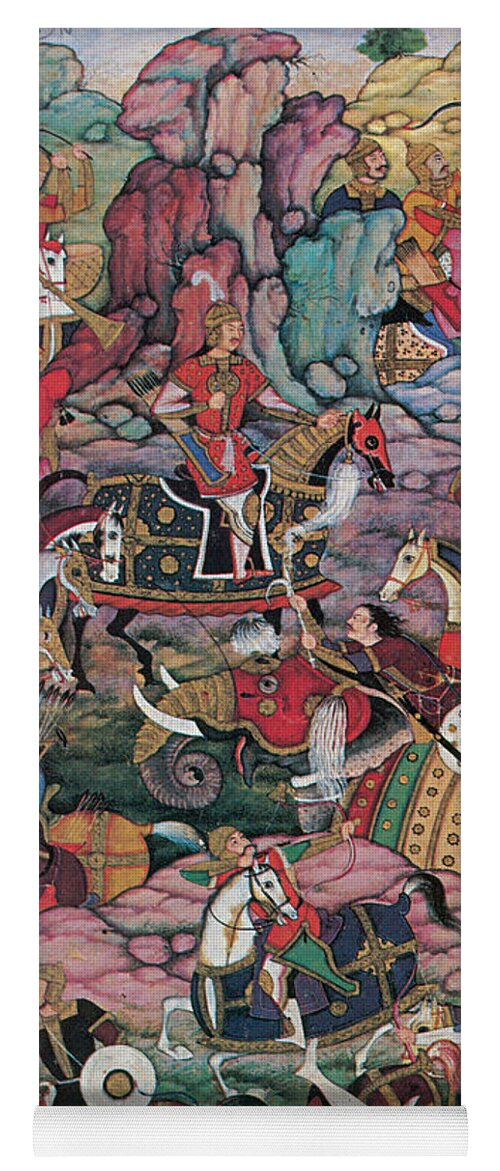The image is a painting depicting a mythological tale, featuring a vivid and surreal scene filled with vibrant colors, predominantly purple and pink hues. The composition is densely populated with various characters and animals, primarily horses, which the majority of the people are riding. The setting appears to be inspired by historical Asia, though it is timeless and lacks specific dating or text.

At the top left, there is a horse adorned in full armor, with a man in a red cloak riding eastward; however, his head is obscured. Above this figure, another man is seen reaching towards an elephant, which is richly bedecked with colorful garb, highlighting its tusks and trunk. Further atop, a second horse and rider are positioned, blending seamlessly into the backdrop alongside two other men, giving a surrealist quality that blurs the lines between the figures and the fantastical elements growing from the ground. These abstract shapes, devoid of real-life equivalents, are red, purple, and blue, and contribute to the otherworldly feel of the painting. 

On the ground, vivid pink rocks are scattered, while the middle of the scene is dominated by an elaborately decorated elephant, asserting the central battle readiness of the characters. Throughout the image, the warriors and their mounts, draped in colorful garments and decorations, evoke a sense of imminent conflict amidst a dreamlike, vibrant landscape. The topmost section of the painting features mushroom-shaped clouds in purples, greens, and reds, further emphasizing the fantastical and richly colored nature of the artwork.